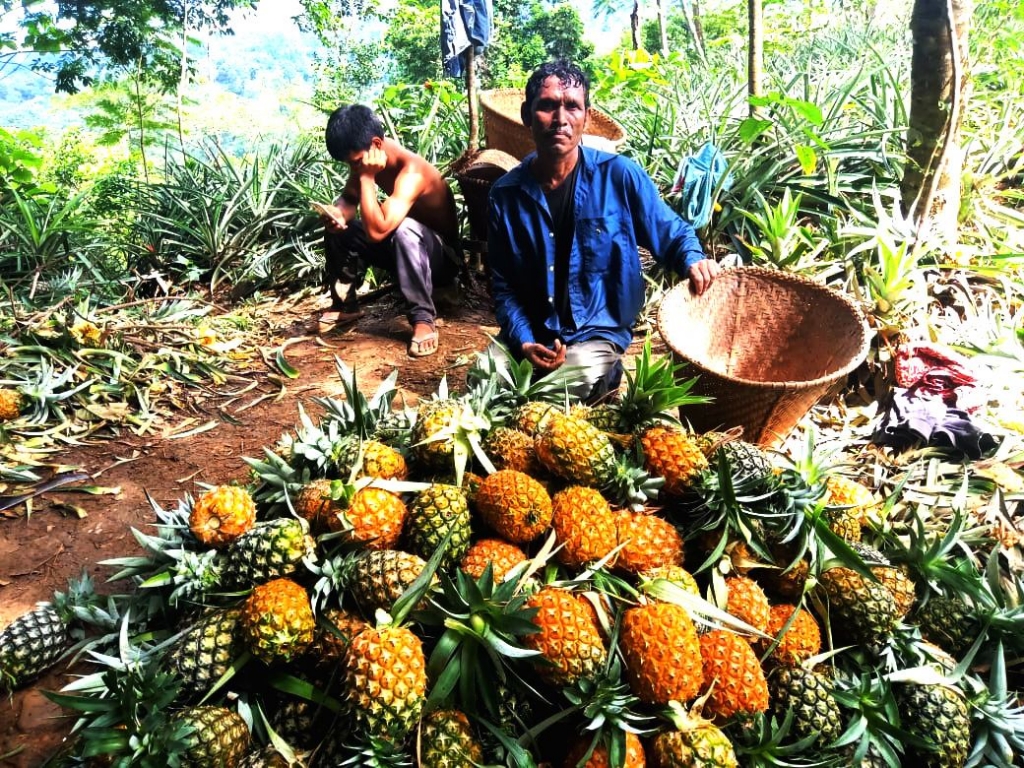The photograph captures an outdoor scene featuring a man and a young boy, presumably engaged in harvesting pineapples. The man, who appears to be of Indian or Polynesian descent, is central in the image, wearing a bright blue shirt and tan pants. His dark hair and tanned complexion are prominent as he holds an empty wicker basket in his left hand. Beside him, to his right, sits a shirtless boy, possibly 10 or 11 years old, wearing gray pants and white flip-flops. The boy has short dark hair and is fixated on a phone or something on the ground with his elbows resting on his knees.

In front of them lies a substantial pile of pineapples, showcasing a mix of green, brown, orange, and yellow hues, all with their leafy crowns intact. The ground around them is scattered with dirt, leaves, and plant debris, adding to the rustic atmosphere. Behind them, a dense backdrop of trees and tropical foliage suggests a lush, verdant environment. The overall scene is bathed in bright, sunny light, further emphasizing the natural setting of this pineapple-harvesting activity.